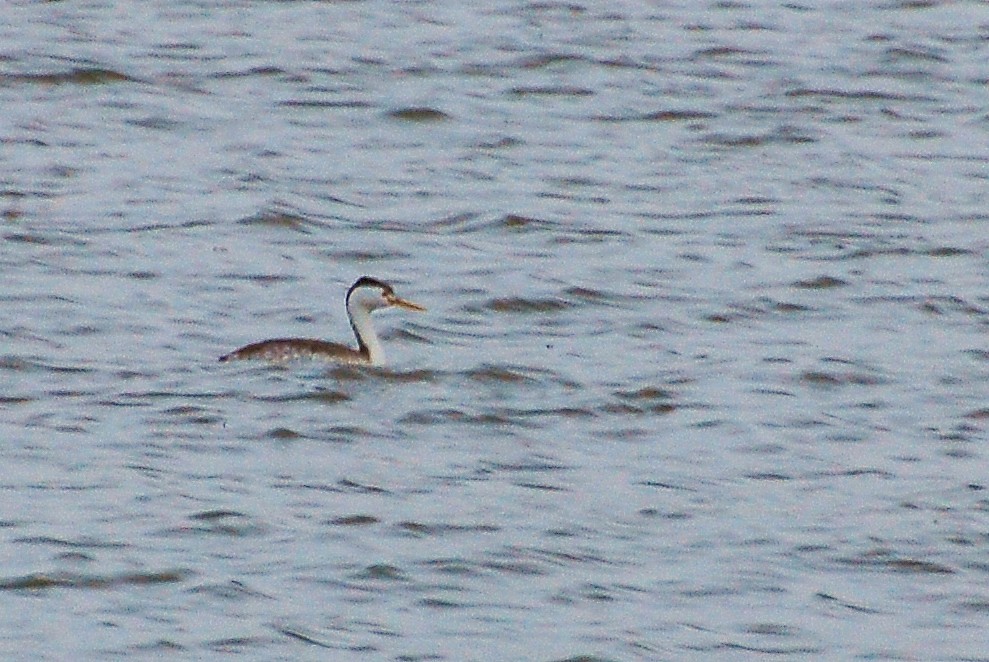The image showcases a bird, most likely a Cochrane, floating serenely on a large, choppy body of water. The bird, distinguished by its long bill, white chest, dark crown, and dark feathers, appears to be gently gliding on the undulating waves, possibly in search of fish. The waters around it are brown and ripple with waves about eight inches high, suggesting it could be either a vast lake or the ocean. The camera perspective is directed downward at the bird, not revealing the horizon but emphasizing the outdoor setting and the wildlife scene. The bird is positioned heading from left to right on a semi-sunny day, though the sky is not visible in the photograph.